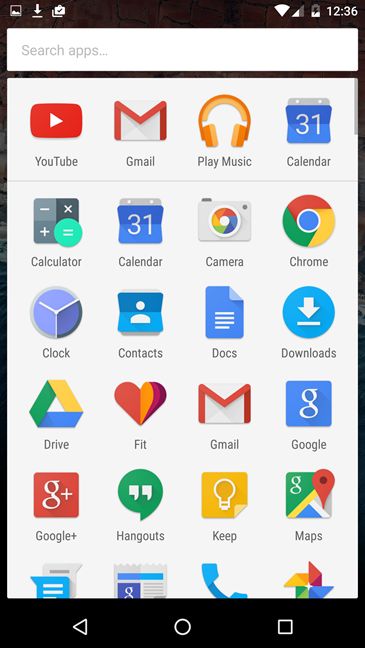The image showcases a screenshot of a smartphone home screen, indicating its functionality within a smart home setup. In the top-left corner, there's a battery icon that is not fully charged alongside a Wi-Fi signal that is not at full strength. The time displayed is 12:36. The home screen is populated with 24 app icons: YouTube, Gmail, Play Music, Calendar, Calculator, Calendar, Camera, Google Chrome, Lock, Contacts, Docs, Downloads, Drive, Fit (with a heart symbol), Gmail, Google+, Hangouts, Keep, Maps (identified by a small red pin), and a multi-colored pinwheel icon. Navigation controls with left arrow, circle, and square symbols are located at the bottom of the screen. The screen is framed by black borders, adding contrast to the vivid display of icons.